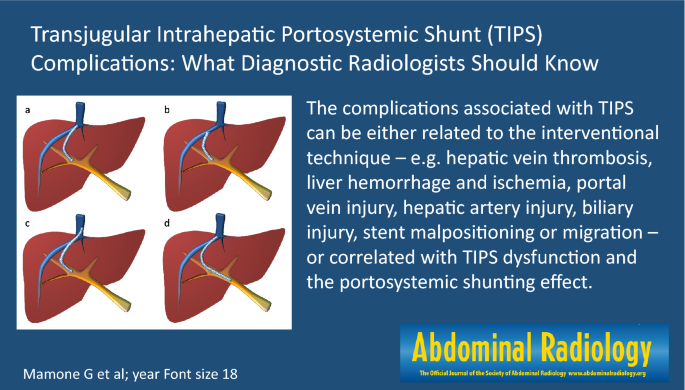The informational graphic features the title "Transjugular Intrahepatic Portosystemic Shunt (TIPS): Complications What Diagnostic Radiologists Should Know" prominently displayed. Set against a blue background, the graphic includes a detailed diagram in the left and left-middle section, illustrating four different pathways of vessels leading through the liver, labeled A, B, C, and D. A citation "Mamon G. et al., year font size 18" is noted below these illustrations. The graphic outlines complications associated with TIPS, including hepatic vein thrombosis, liver hemorrhage and ischemia, portal vein injury, hepatic artery injury, biliary injury, and stent malpositioning or migration. It also discusses complications related to TIPS dysfunction and portosystemic shunting effects. In yellow text on the bottom right, it states, "Abdominal Radiology, the official journal of the Society of Abdominal Radiology," accompanied by a website URL.